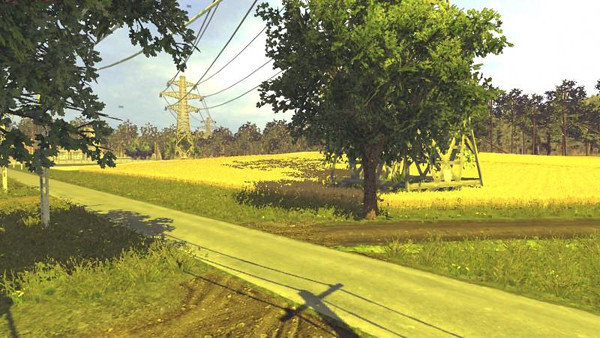This seemingly surreal image depicts a scenic outdoor landscape, which may be either a meticulously painted scene or a digitally rendered artwork. In the foreground, a dirt road, tinted with a peculiar yellow hue, stretches forward. To the right of the road stands a solitary tree with rugged brown bark and a lush green canopy, providing a stark contrast against the open space.

In the distance, a grove of trees can be seen, their shadows hinting at the bright sun overhead. Adding to the composition is an array of large three-pronged metal electrical towers, which cast long shadows across the terrain. The presence of one wooden electrical pole with its shadow further emphasizes the sunlit setting.

Off on the horizon, a faint structure, possibly a house, emerges, seamlessly blending into the dreamy and somewhat enigmatic atmosphere of the scene.